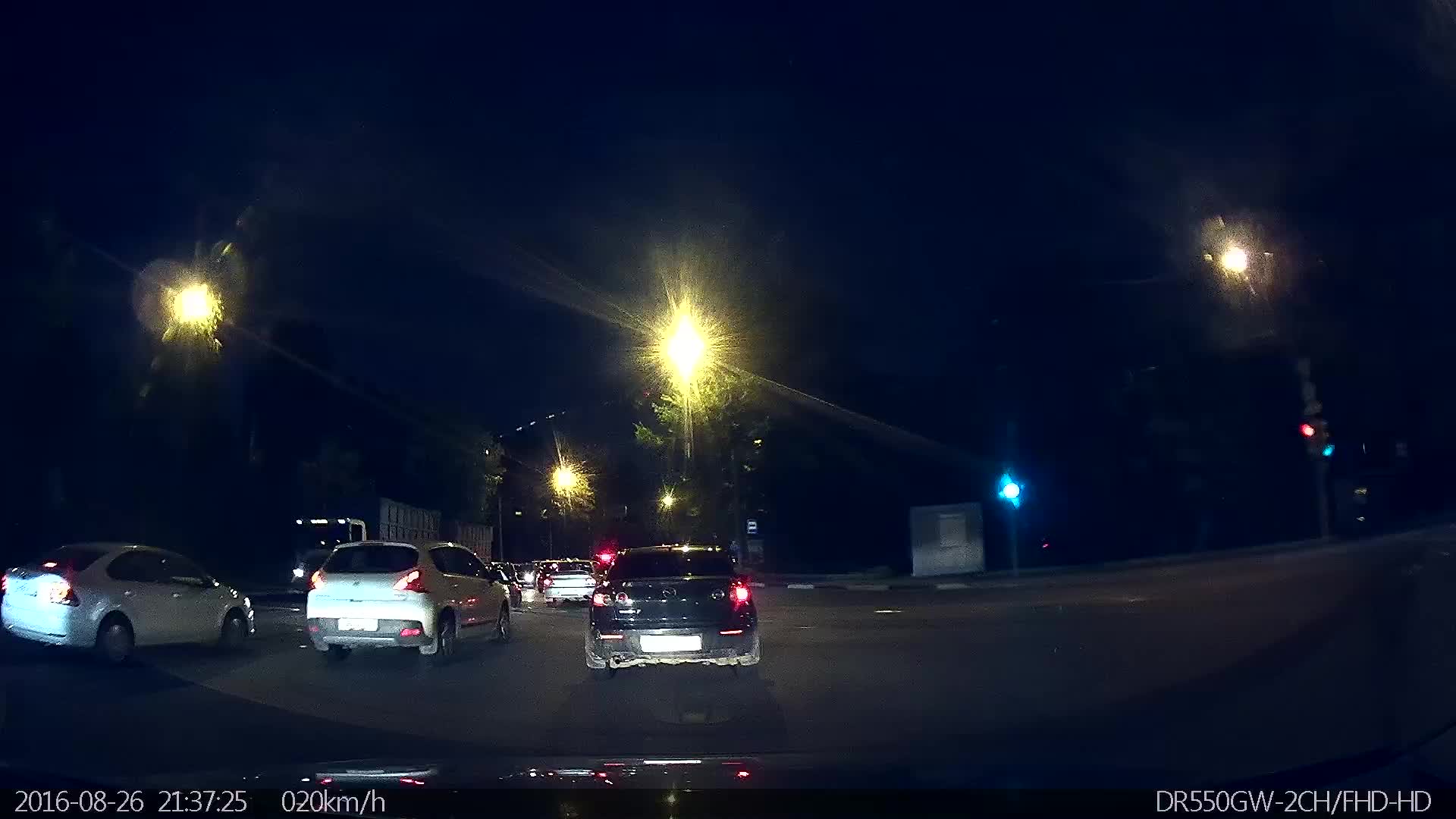Captured during the night, this image depicts a street scene from the perspective of a vehicle in motion. The overall atmosphere is exceptionally dark, suggesting a lack of street lighting beyond what the vehicle headlights provide. In the lane directly ahead, a black car has come to a stop. Meanwhile, in the two adjacent lanes to the left, there are small, light-colored cars progressing through a yellow traffic light. The bottom of the image features a timestamp and various data codes: it is marked with the date "August 26, 2016," the time "21:37:25," and the speed "20 KM/H." Additional alphanumeric codes such as "DR550GW-2CH/FHD/HD" are also visible, likely indicating details related to the capturing device or image metadata.